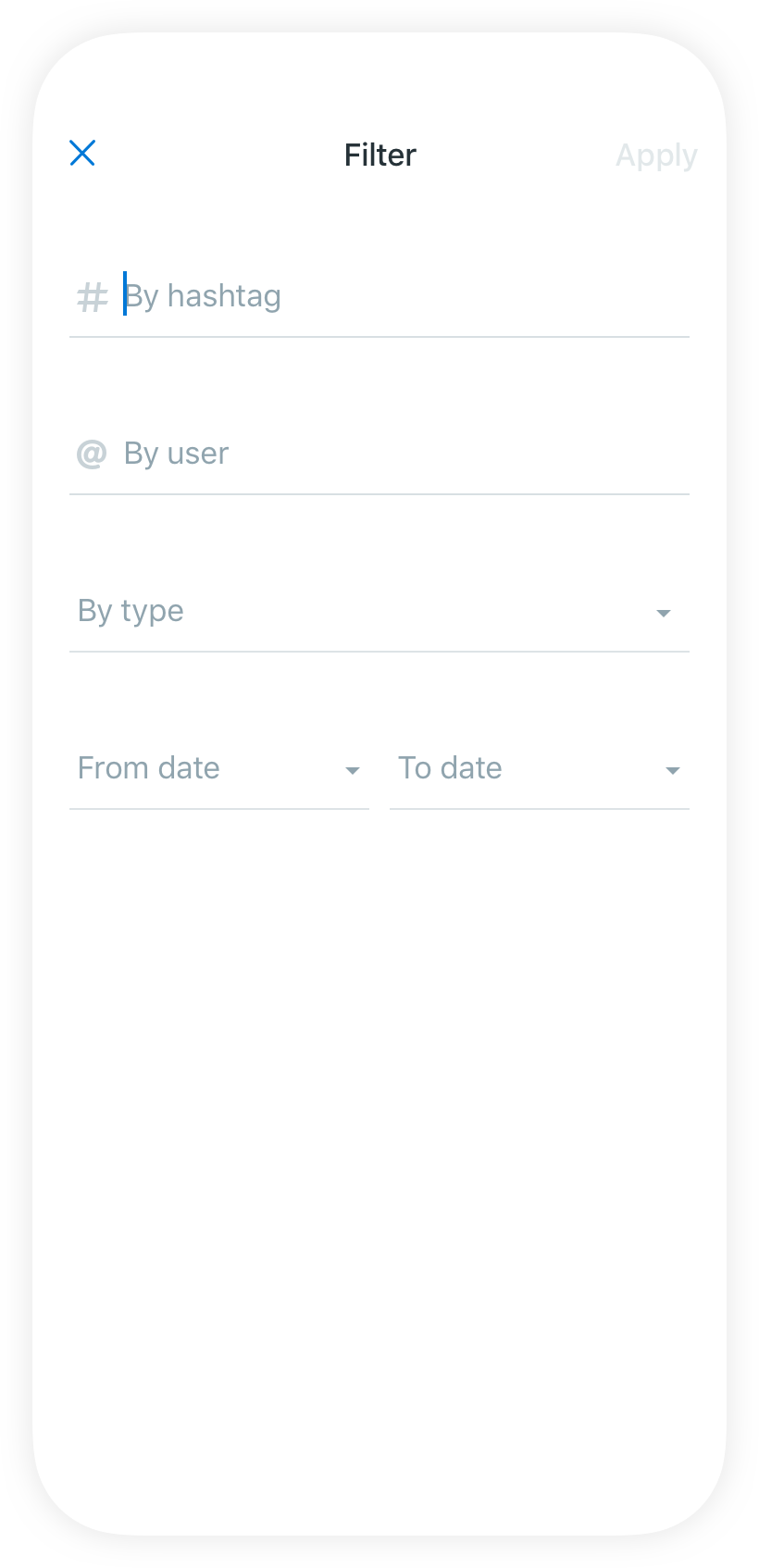This image is a screenshot from a cell phone. The display has rounded corners, which is characteristic of many modern phones. The background of the image is entirely white, and there is a subtle shadow effect around the edges, particularly in the corners.

In the upper left corner, though not exactly at the edge, there is a blue "X" icon. At the top center of the screen, the word "Filters" is displayed prominently. On the upper right corner, there is a dull gray "Apply" button.

Further down, the screen displays various input lines. First is the input line titled "By Hashtag," followed by "By User" as another input line beneath it. Next, there is an input line labeled "By Type." At the bottom of these input fields, there are two additional fields labeled "From Date" and "To Date" respectively.